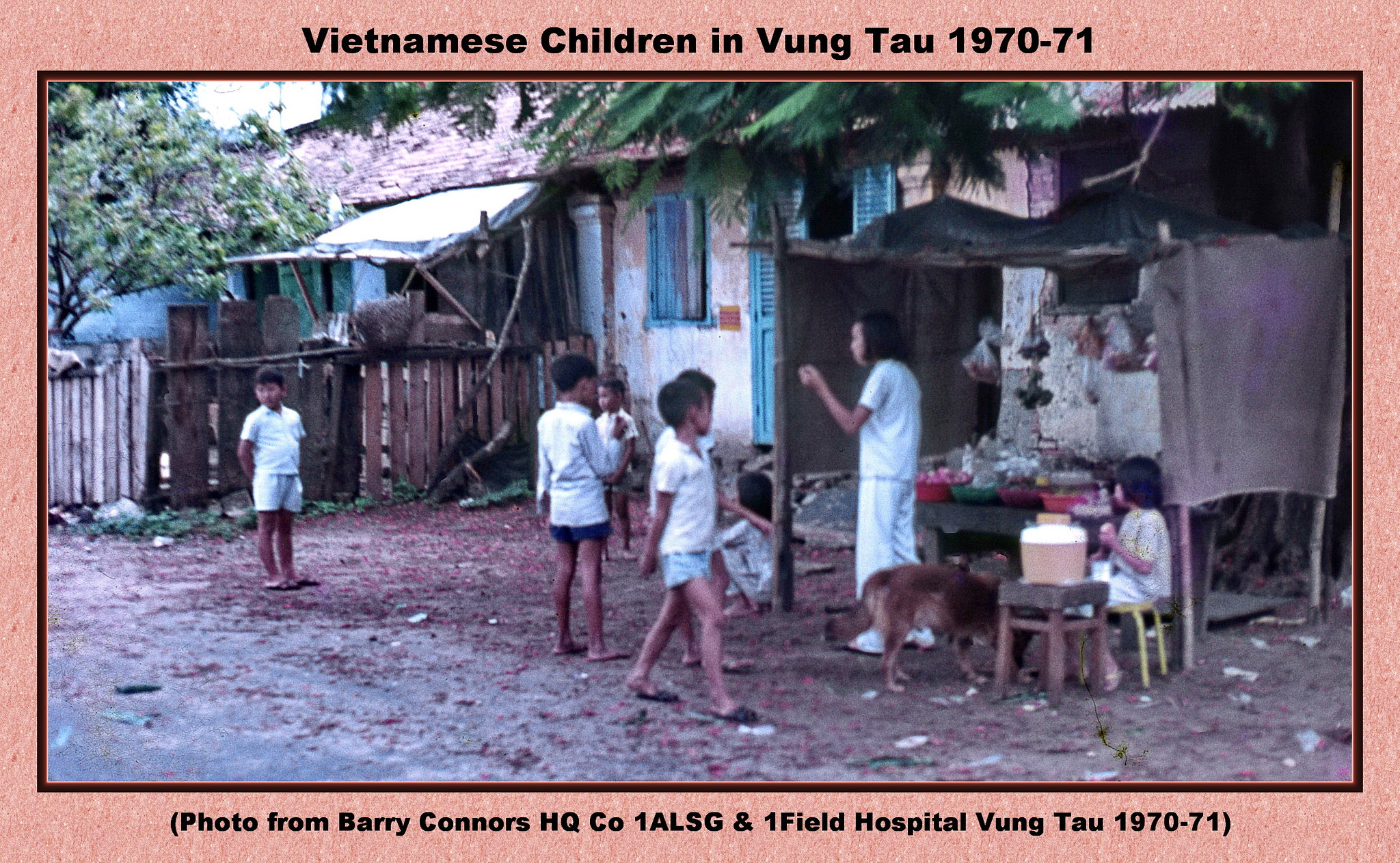The image, titled "Vietnamese children in Vung Tau 1970-71," features a group of seven to eight children and a woman, likely their mother, standing outside a small, dilapidated house. They are dressed in shorts, T-shirts, and some sandals, indicative of the warm weather. The house, resembling a shack, appears run-down and possibly covered with tarps and other makeshift materials, rather than solid wood. The ground around the house is a mix of dirt, garbage, and sparse vegetation, with some greenery and trees visible in the upper parts of the image. A makeshift tent-like area made from cloth draped over posts, possibly holding food, is situated to the right, while an improvised awning created from sticks and materials extends from the house. A dog is also present among the children. The photograph has a pink, peachy border and includes a caption at the bottom mentioning it is a photo from Barry Connors, HQ CO 1 ALSG and one field hospital Vung Tau, 1970-71.